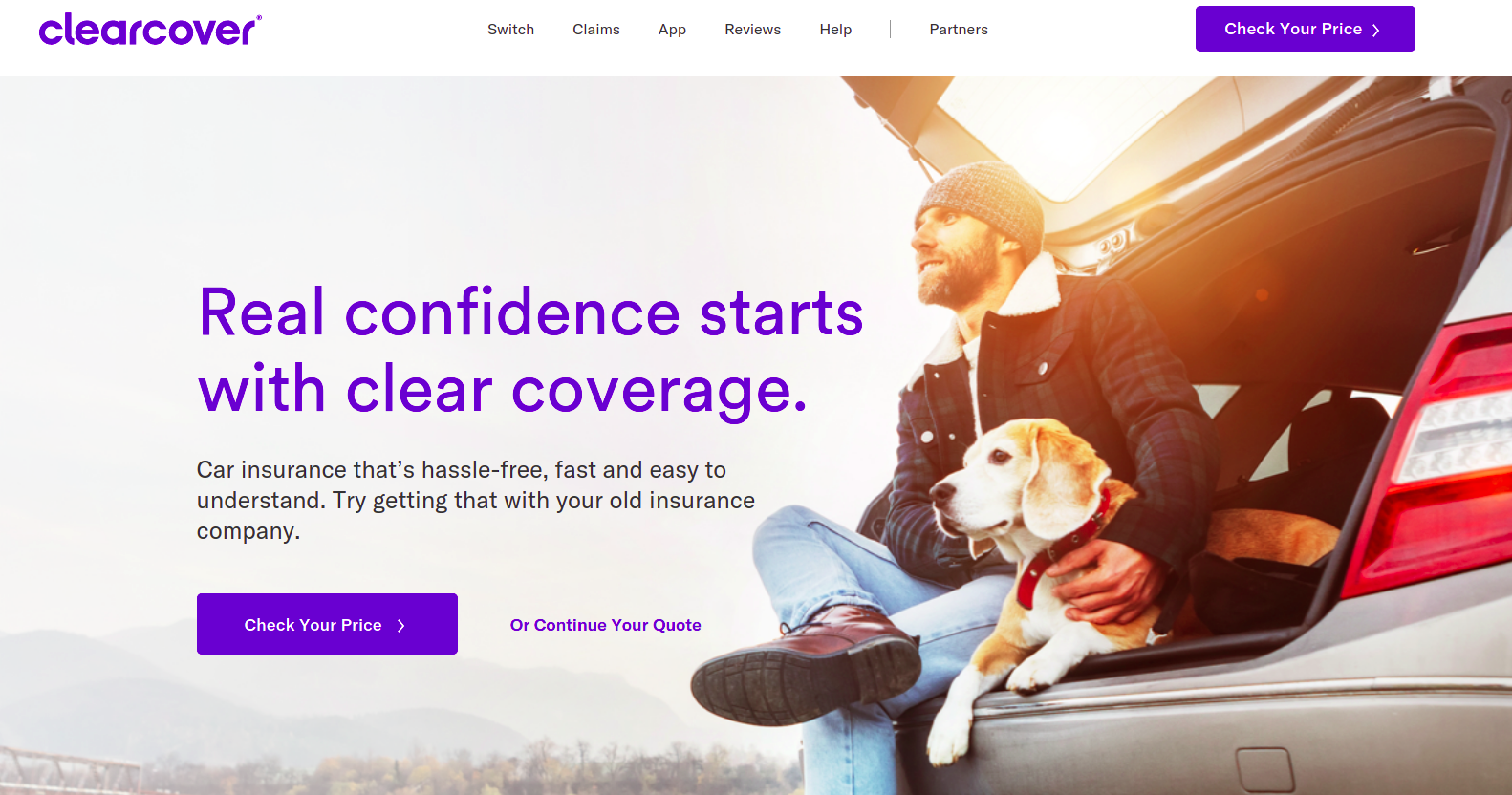The image features a website interface with a minimalist and clean design. At the top, the text "clearcover" is displayed in lowercase purple letters against a white background. Below this, there is a navigation bar with the options "Switch," "Claims," "App," "Reviews," and "Help," followed by a vertical line and the word "Partners." On the right side of the navigation bar, there is a button with a red or purple background and white text that reads "Check Your Price," featuring a right-pointing arrow.

The midsection of the image transitions to a gray background, depicting an outdoor scene with a person sitting in the trunk of a car, a mountain or hill area in the distance, some trees, and what appears to be part of a bridge. The environment suggests a serene and natural setting. Superimposed on this background, the text "Real Confidence starts with clear coverage" is displayed in purple, with a subtext in black print saying, "Car Insurance that's hassle-free, fast, and easy to understand. Try getting that with your old insurance company."

At the bottom, a purple band features the text "Check Your Price" with a right-pointing arrow, while outside of this band in purple print, it reads "or check or continue your quote." Further, there's an image of a man sitting in the open trunk of a car, accompanied by a Beagle dog, adding a personal and relatable touch to the scene.